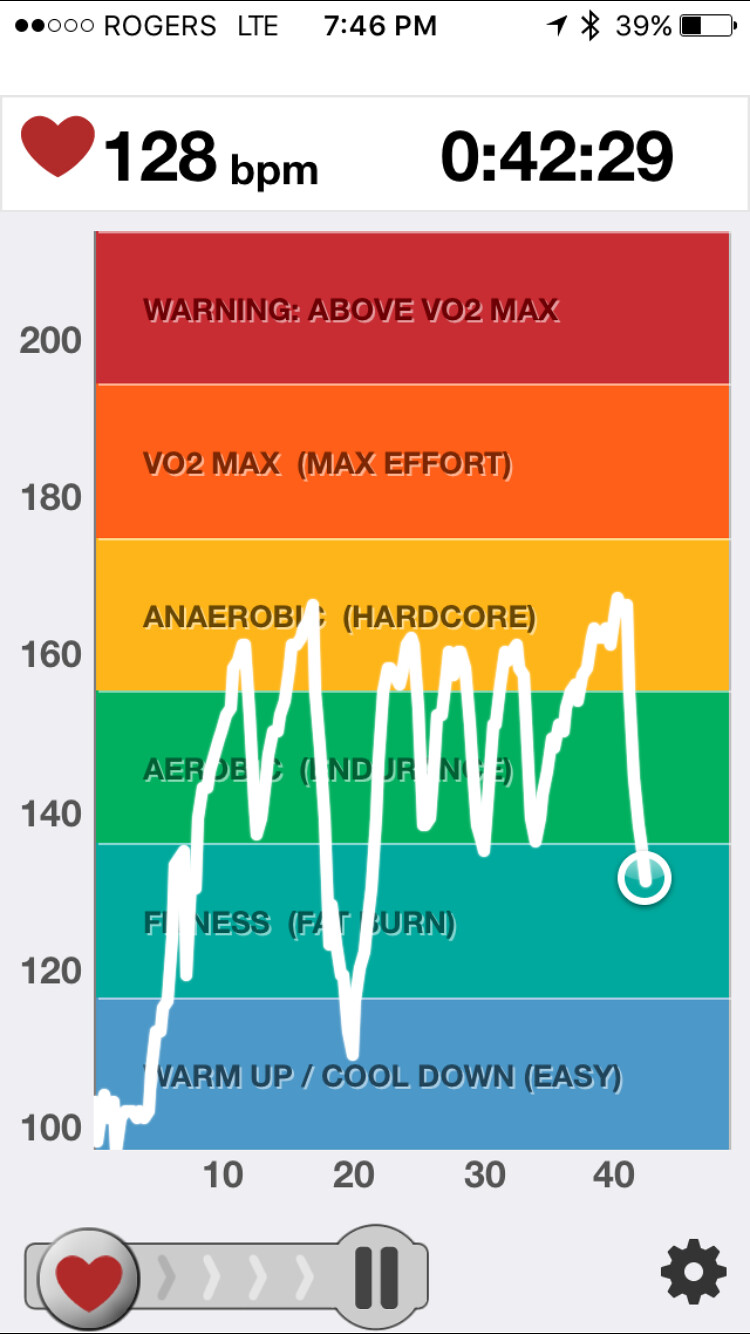The screenshot captures a white-background mobile screen at 7:46 PM, showing Rogers LTE with 39% battery and two of five signal bars. The screen features a fitness app with a red heart icon indicating the user's heart rate at 128 BPM, alongside a timer reading 0:49:29. A chart tracks the heart rate over time, displaying fluctuating values from 100 to 160 BPM, and categorizes different heart rate zones: 100 (warm-up/cool-down/easy), 120-140 (fitness/fat burn, green), 140 (aerobic/endurance, light green), 160 (anaerobic/hardcore, yellow), 180 (VO2 max/max effort, orange), and 200 (above VO2 max, red warning). A waveform representing the heart rate data traverses these zones, illustrating periods of higher intensity and rest. The lower left corner features a draggable slider with a heart logo and progress arrows, while the bottom right shows a settings icon.